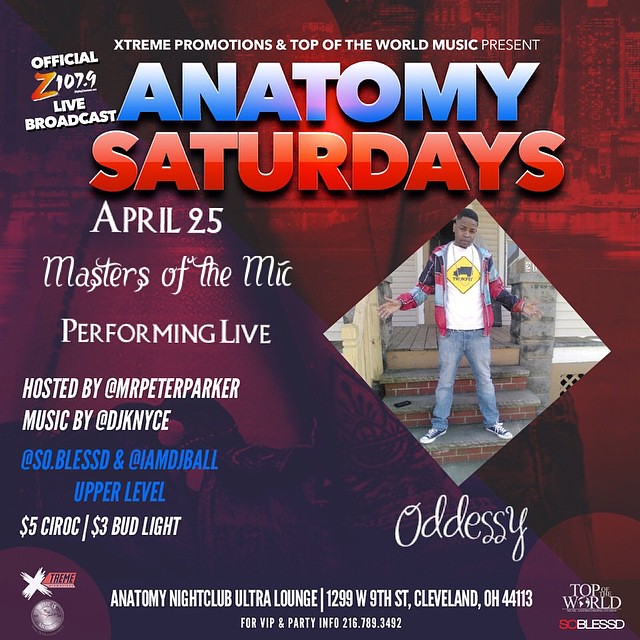The promotional poster for the Anatomy Saturdays nightclub event is vibrant with prominent red and black hues. Dominating the poster is an image of a young man, possibly in his early 20s, wearing a blue and red flannel jacket over a white shirt with a yellow diamond insignia, blue jeans, and white and black sneakers. He is framed within a diamond-shaped border, standing on brick-lined steps against a dark red background. 

The text on the poster offers detailed event information: "Extreme Promotions and Top of the World Music present Anatomy Saturdays." It announces an official Z107.9 live broadcast on April 25th, featuring "Masters of the Mic performing live," and is hosted by Mr. Peter Parker with music by DJ K Nice. Additional mentions include services by So Blessed and I Am DJ Bo, located on the upper level. Offering notable drink specials, the event includes $5 Ciroc and $3 Bud Light. The venue is the Anatomy Nightclub Ultra Lounge, located at 1299 West 9th Street, Cleveland, Ohio, 44113, with VIP and party info available at 216-789-3492. The poster also includes branding elements with "Top of the World" in the bottom right corner and "So Blessed" in the top left corner.